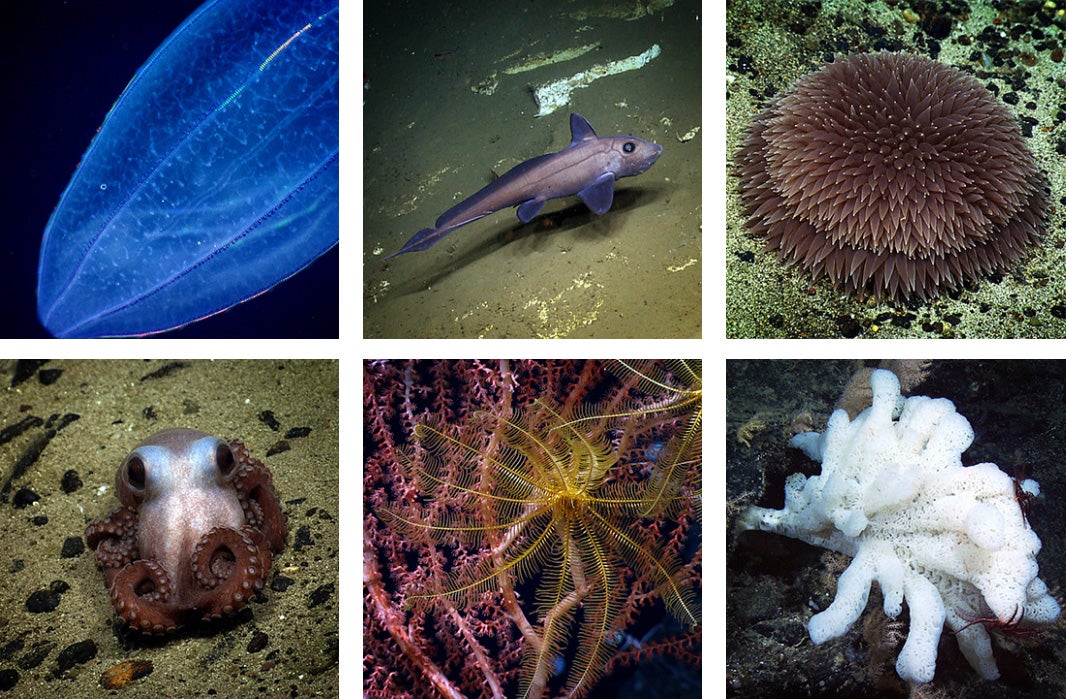This image set consists of six detailed close-up photos of various sea creatures arranged in a grid with three photos on the top row and three on the bottom row. 

In the upper left, there's a translucent, bright blue organism with a jellyfish-like appearance. Next to it, in the upper middle, a fish is captured resting on a dark brown, slightly greenish ocean floor, its single black eye directed towards the camera. The upper right features what seems to be a maroon-brown sea anemone, fanned out like an underwater flower.

On the bottom left, a small brown octopus is shown on the sea floor, seemingly interacting with the observer. The bottom middle showcases pink coral adorned with a yellow, plant-like creature that has many limbs, resembling an underwater spider. Finally, the bottom right image displays a white piece of coral set against a backdrop of rocks, possibly part of a larger coral reef.

These diverse and vibrant photographs highlight the rich variety of life found beneath the ocean’s surface.